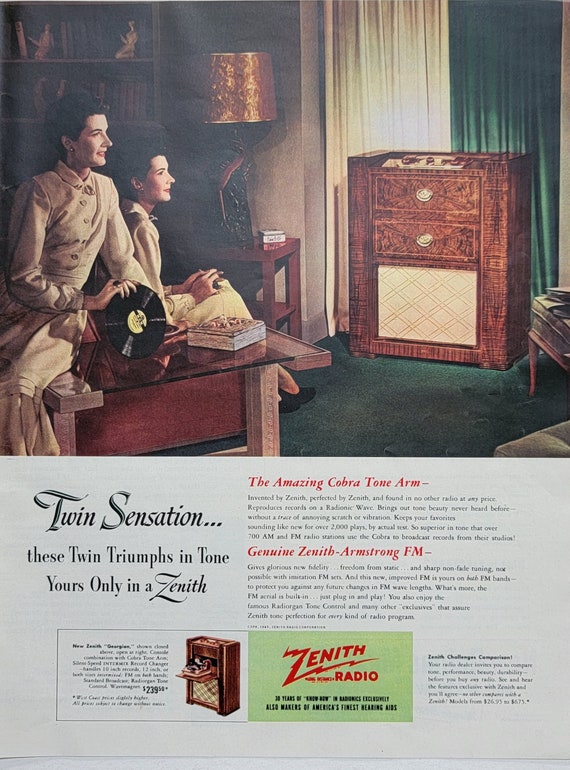This detailed vintage advertisement for a Zenith Radio, likely from the early 1900s, features a meticulously illustrated living room scene on the upper half. Two women, dressed in tan jackets, sit in front of a wooden, wood-grain Zenith radio with a lighter-colored speaker panel. Their setting includes green carpeted floors, dark and white drapes, a brown dresser, a lamp, and a bookshelf. The lower part of the advertisement is filled with promotional text: "Twin Sensation - These twin triumphs in tone, yours only in a Zenith." Additional highlighted features include "The Amazing Cobra Tone Arm" and "Genuine Zenith Armstrong FM." At the very bottom, within a designated box, the price of the radio is listed as $239.14.